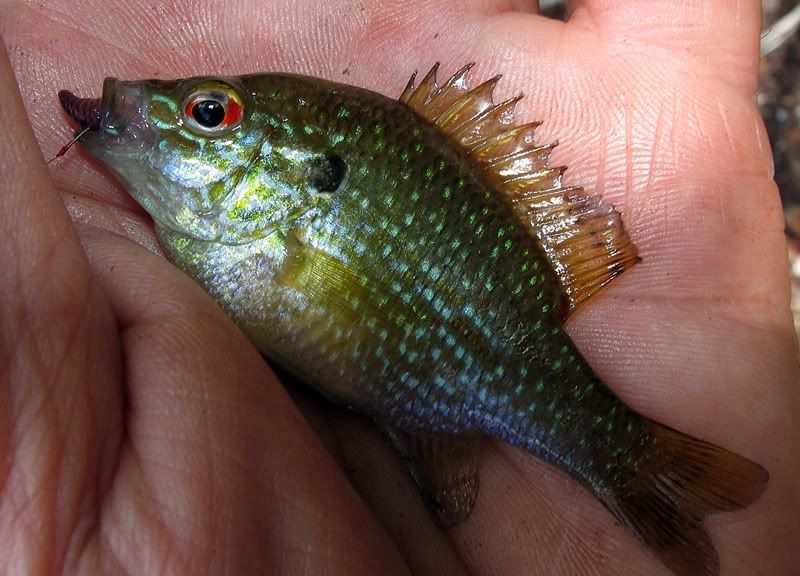In this highly detailed close-up image, a small, vividly colored fishing lure resembling a fish rests in the palm of a Caucasian person's hand. The lure, no more than an inch long, features a shiny green body with white specks and intricate detailing, including a black-centered red eye, a gray mouth with a hook presumably attached, and a gold-orange fin that extends along its back. The close proximity of the shot reveals the texture of the person's skin in great detail. Over the center of the image is a watermark from the photo hosting service PhotoBucket, inscribed with "Photo Bucket" in white letters and surrounded by numerous circular designs, while a transparent gray banner across the lower third displays the text, "Protect more of your memories for less." The confluence of vivid colors—green, red, gold, white, and more—creates a visually striking composition.